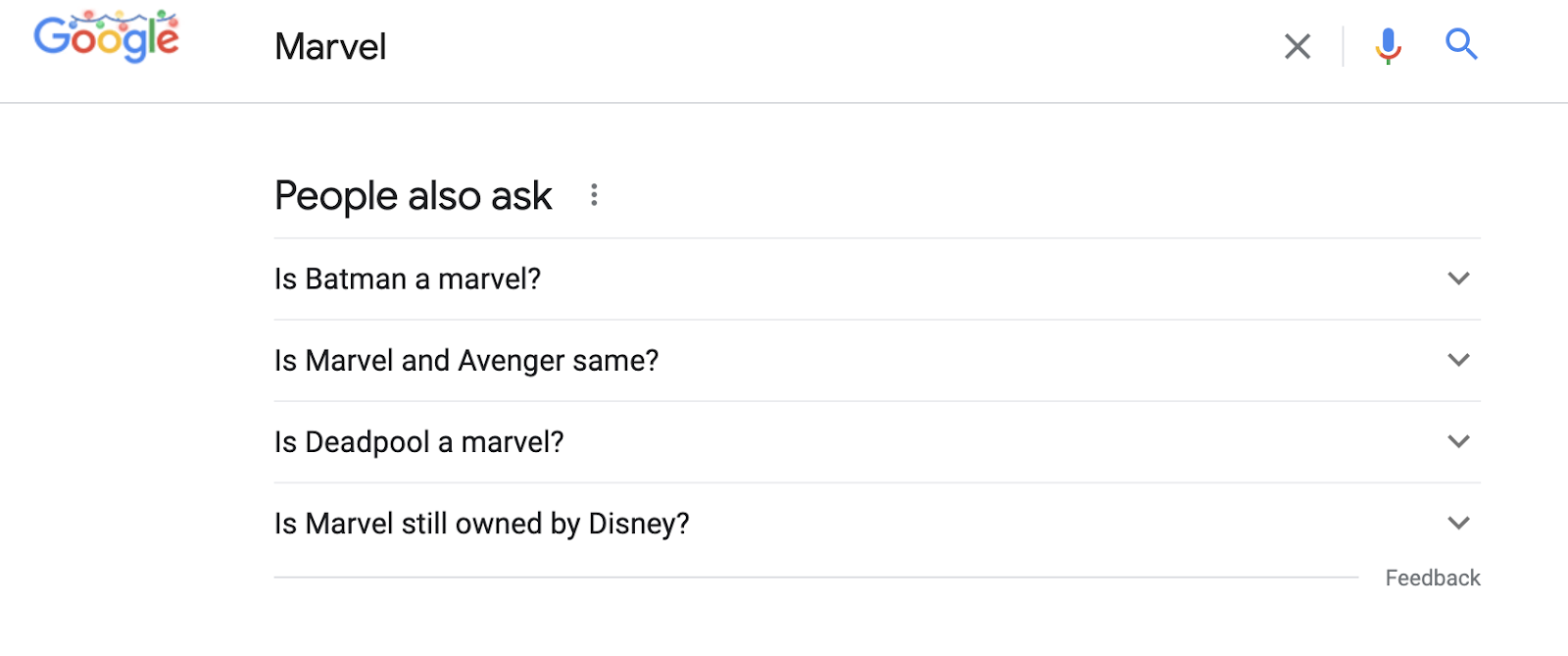This image captures a Google search results page with the query "Marvel" entered in the search field. Prominently displayed below the search bar are a series of "People also ask" questions, including: "Is Batman a Marvel?", "Is Marvel an Avenger?", "Is Deadpool a Marvel?", and "Is Marvel still owned by Disney?". In the top right corner, the close button is visible, flanked by the voice search button and the search button. At the bottom right, there's a feedback link. The text on the page is a mix of blue, red, yellow, and black, all set against a clean, white background, maintaining Google's typical minimalist design.